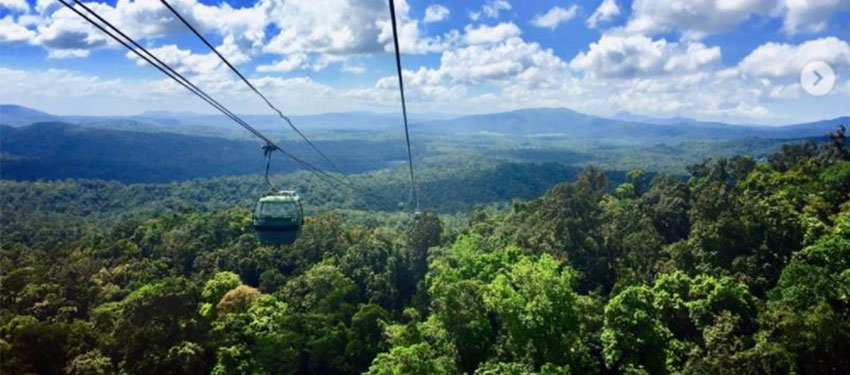The photograph showcases a dark green cable car descending along an extensive cable that stretches high above a densely packed, lush forest. The canopy of the forest below is filled with tall, large trees in varying shades of green, giving off a jungle-like vibe. The forest extends outward, transitioning into emerald green hills that rise and turn into mountains in the distance. The sky above is a vibrant blue, scattered with fluffy, cotton-like clouds casting shadows onto the forest below. In the distance, the mountains appear bluish and span for miles, creating a serene and expansive landscape. The photo captures a beautiful day, with perfect weather and a picturesque scene of nature.